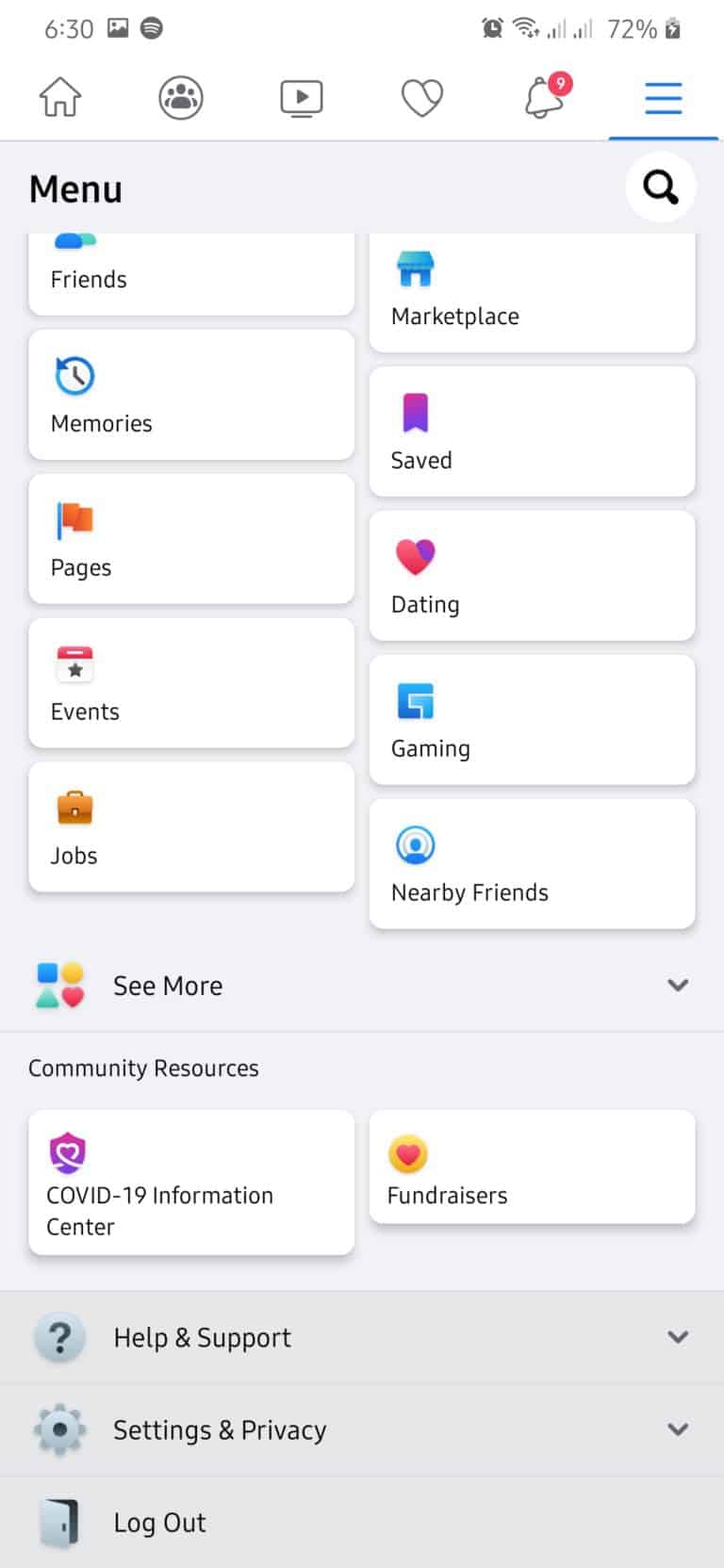At the top of the image, there is a navigation bar featuring several icons: a home symbol, a people symbol, a video symbol, a heart symbol, a bell symbol, and three horizontal bars. Below this bar, a horizontal line separates it from the main menu items, which include a "Menu" label to the right of a magnifying glass icon.

Underneath this are tabs labeled: Friends, Marketplace, Memories, Saved, Pages, Dating, Events, Gaming, Jobs, and Nearby. These tabs are presented in a horizontal layout.

Below these tabs, a dropdown menu labeled "See More" is indicated by an arrow pointing downwards. To the left of "See More," there are four colored shapes: a blue square, a gold circle, a blue triangle, and a red heart, also lined up horizontally.

Under another dividing line, the section labeled "Community Resources" appears. Below this section, there are two boxes. One box is for the "COVID-19 Information Center," and the other is for "Fundraisers."

Beneath these boxes are two more dropdown menus: "Help and Support," marked with an arrow pointing down, and "Settings and Privacy," also marked with an arrow pointing down. At the bottom of the menu, there is a third box labeled "Log Out."

The background features a gray color. To the left side of the interface, there are additional symbols including a question mark, a cogwheel, and a door, corresponding to the icons seen in the menu tabs. Each tab icon is detailed further: the COVID-19 Information Center has a purple heart on a shield, Fundraisers has an orange heart inside a yellow circle, Events has a calendar, Pages has a flag, Marketplace has a small stall, Saved has a bookmark, and Dating has a heart icon.